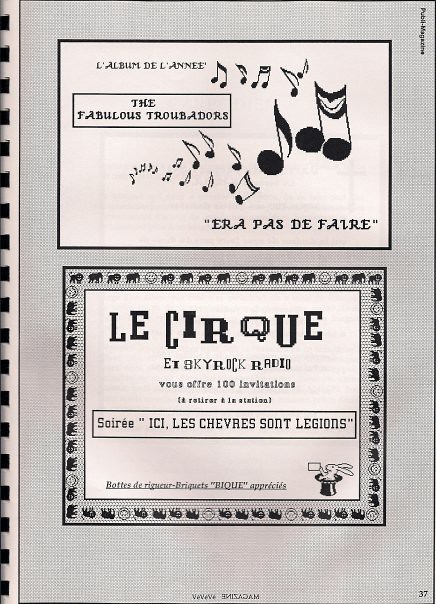The image appears to be the cover of a vintage book or booklet with a spiral binding on the left, featuring black square intervals. The background is a grey burlap texture. At the top, there is a white rectangular box with a black border containing French text: "L’Album de l’Année." Adjacent to this, a collection of musical notes curves from the right side and back around to the middle of the page.

Below the main title, it says "The Fabulous Troubadours." In the bottom right corner, the phrase "Ere pas de faire" appears in quotes. Below this is another rectangular box with black borders containing images of animals, including elephants and lions, around its inner border. Inside this box, the headline "LE CIRQUE" appears in white letters with a magazine-like font, followed by the subheading "ET Skyrock radio" and a line stating "VOUS OFFRE 100 invitations."

Further down, there is a banner with the text: "SOIRÉE 'ICI, LES CEVAES SONT LÉGIONS.'" The bottom part of the image is somewhat blurry but seems to include a footnote in a less clear font. In the extreme lower right, there is an illustration of a rabbit emerging from a top hat, holding a card. The center bottom part has some illegible, possibly reversed text, resembling the words "magazine" printed in reverse.